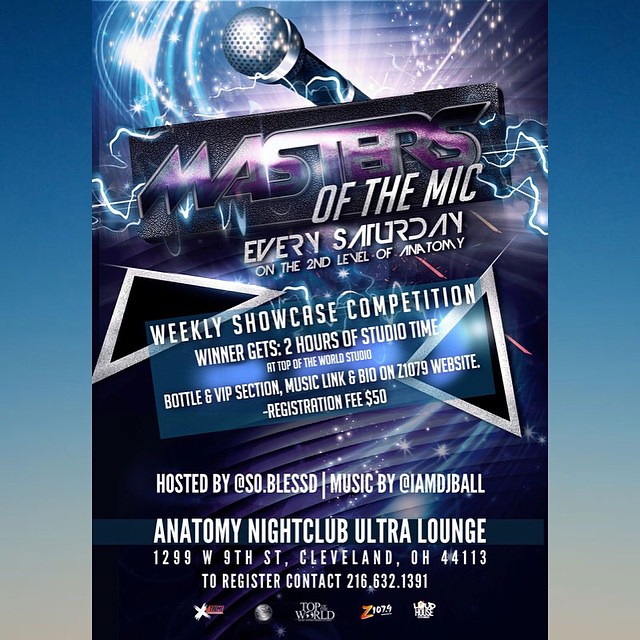The promotional flyer for the event features a striking blue gradient border that transitions from dark blue at the top to light gray at the bottom. The main background is dominated by dark colors, primarily black and dark blues. At the top, multiple lines with cartoon-like stars and lightning bolts emanate from a central logo: a black rectangle with purple lettering that reads "Masters," crowned by silver text "of the Mic," with a cartoon 3D microphone slightly poking out from behind.

Just below this central logo, silver text announces: "Every Saturday on the Second Level of Anatomy." Centrally located on the poster, a see-through blue rectangle with white font provides additional details. It promotes a weekly showcase competition held at Anatomy Nightclub Ultra Lounge, located at 1299 West 9th Street, Cleveland, Ohio 44113. The flyer also mentions the registration fee of $50, adds that the winner will get two hours of studio time at Top of the World Studio along with a bottle and VIP section.

Further details include the event being hosted by prominent figures, with music by DJ Ball. For more information, it directs participants to the Z1079 website and provides a registration contact number: 216-632-1391.